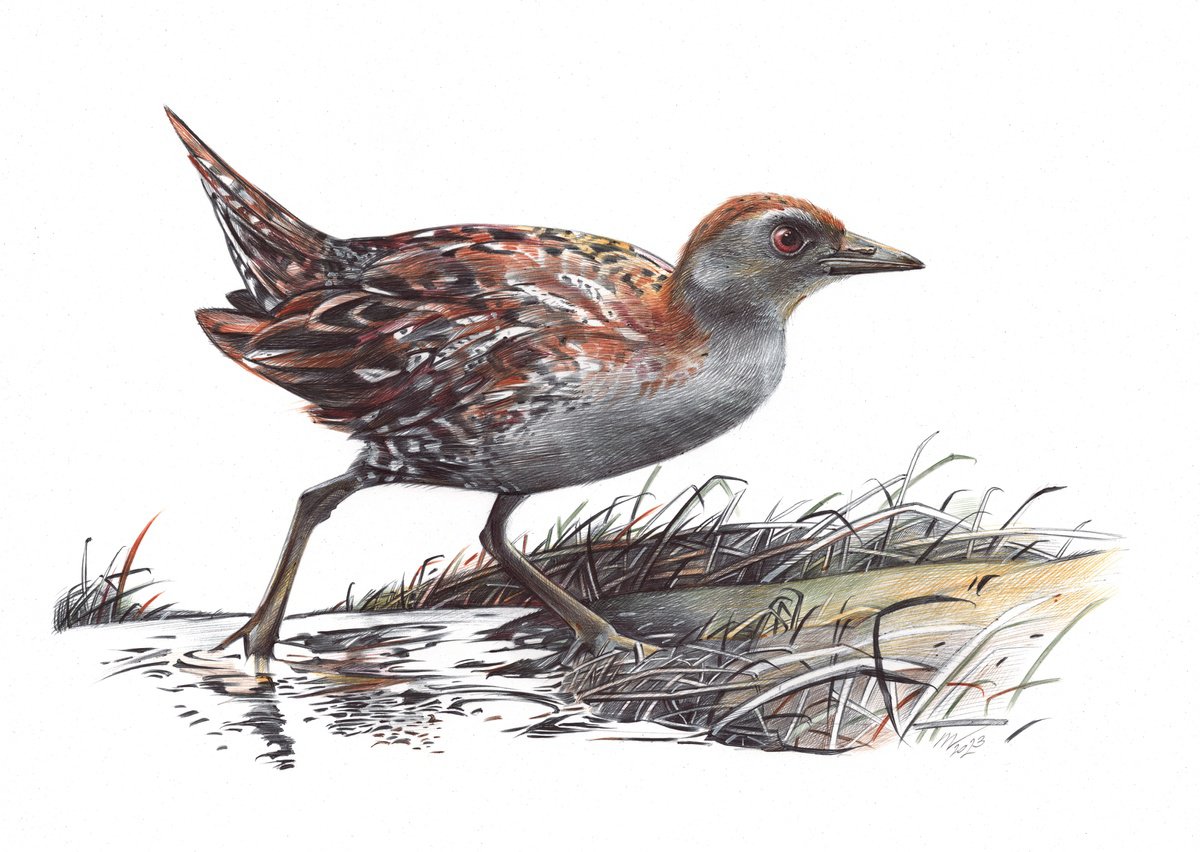This artwork depicts a medium-sized bird wading through marshy water, transitioning onto land. The bird has strikingly long legs and a predominantly gray body, accented with an array of feathers in red, white, and black. Its right side is visible, showcasing its pointed, dark gray beak and vivid red eyes. The bird’s tail feathers taper into a point, while its underside appears whitish-gray. The slightly brownish-yellow feathers at the top transition to a dark reddish brown toward the tail. 

The scene captures the bird stepping out of the dark gray water, creating ripples around its legs. Surrounding the bird, there are tall, whitish-brown and gray grasses that emphasize the marshland setting. The land beneath the bird’s foot is a blend of dark brown and green, suggesting fertile, wet earth. The sky and distant background of the painting are starkly white, drawing attention to the vibrant details in the foreground.